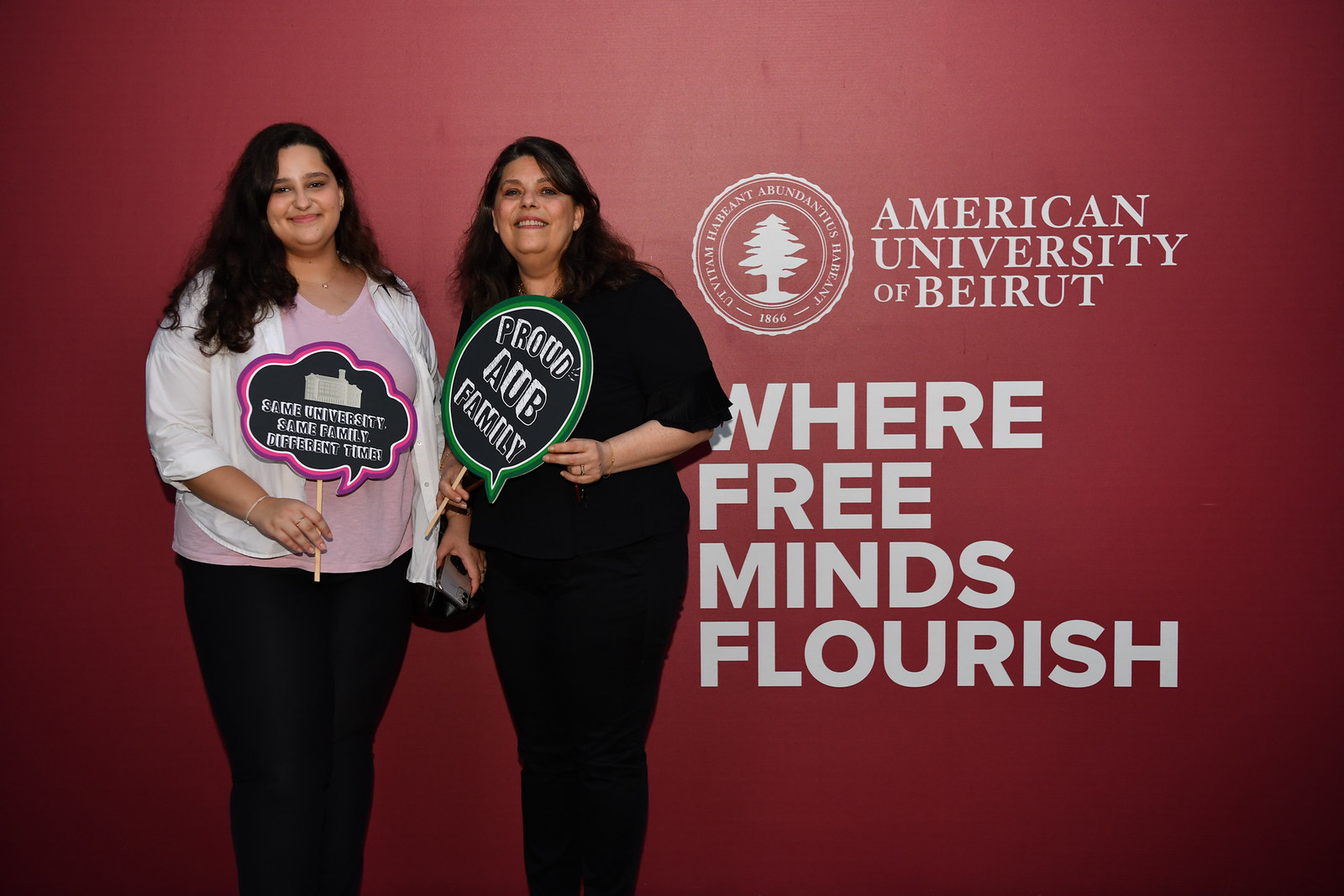In this vibrant image, two smiling women stand in front of a large red banner adorned with the American University of Beirut's logo, which features a tree and the year 1866, along with the motto "Where free minds flourish" in white text. The woman on the right has long brown hair with hints of gray and is dressed entirely in black. She proudly holds a sign with a green-trimmed speech bubble that reads "Proud AUB Family." The woman on the left sports long, curly black hair and is dressed in black leggings, a pink shirt, and a white blouse. She holds a sign with a purple-outlined speech bubble that states "Same University, Same Family, Different Time." Both women are positioned slightly to the left of the image and share a backdrop that prominently features the name of the university.